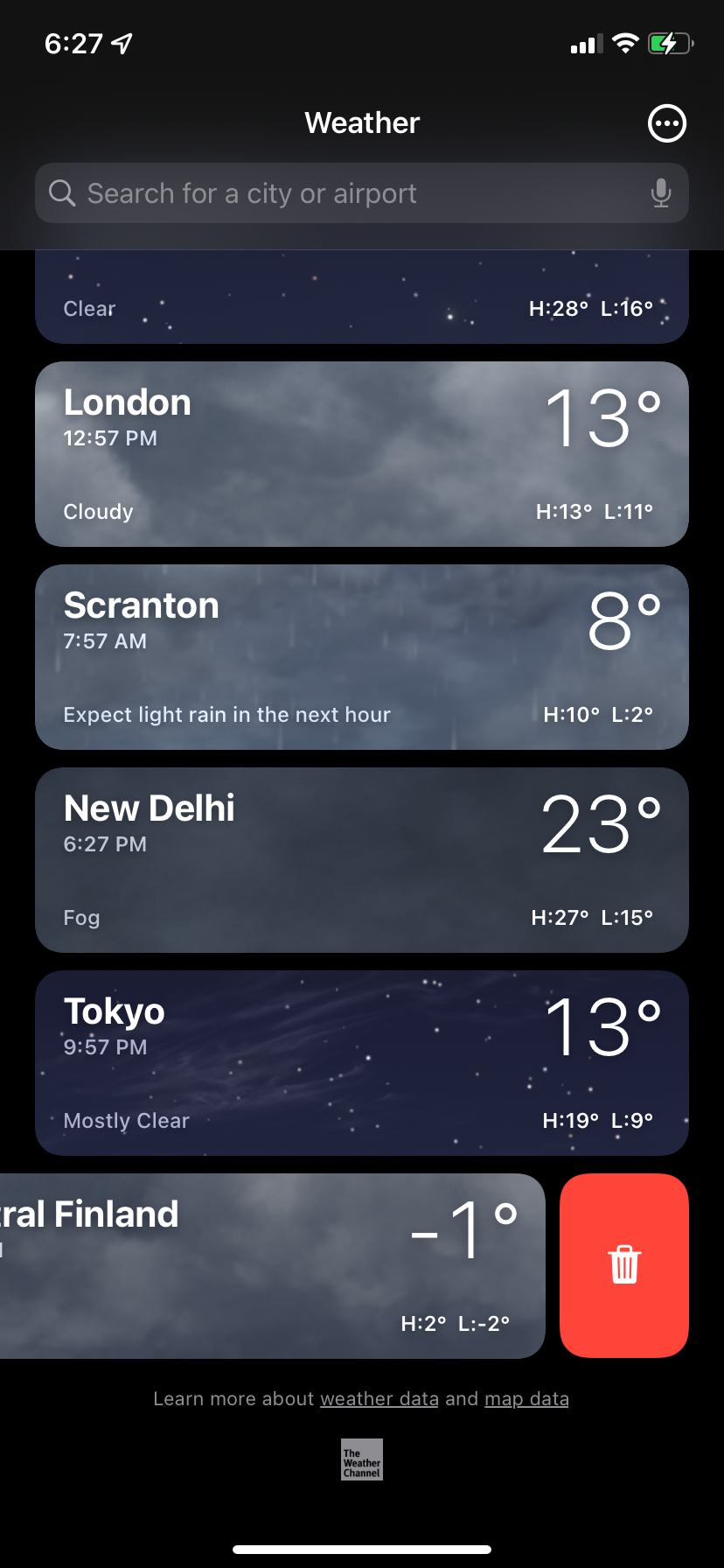This image is a screenshot of weather information displayed in a mobile application. The background is predominantly black. At the top header, there is centered white text reading "Weather," flanked on the right side by a white outlined circle containing three horizontally-aligned white dots. Just below the header, there is a medium gray search bar with light gray icons and text. On the left side of the search bar, there's a magnifying glass icon, followed by the text "Search for a city or airport." Positioned on the far right of the search box is a microphone icon.

Underneath the search bar, a thin light gray line separates it from the weather information below, which is presented on a black background. Each weather information panel features an image of the sky as its background and is framed by a rectangle with rounded corners. These panels are slightly separated from one another by strips of the black background.

1. The first panel, only partially visible, shows a starry sky with a slight blue tinge. In the bottom left corner, there is white text that says "Clear." In the bottom right, it indicates "H: 28° L: 16°."

2. The second panel, for London, displays the following information: 
   - Top left: "London"
   - Beneath it, in smaller text: "12:57 PM"
   - Top right: "13°"
   - Bottom left: "Cloudy"
   - Bottom right: "H: 13° L: 11°"

3. The third panel, for Scranton, includes:
   - "Scranton"
   - "7:57 AM"
   - "8°"
   - Text in the center: "Expect light rain in the next hour."
   - Bottom right: "H: 10° L: 2°"

4. The fourth panel, for New Delhi, shows:
   - "New Delhi"
   - "6:27 PM"
   - "23°"
   - "Fog"
   - Bottom right: "H: 27° L: 15°"

5. The fifth panel, for Tokyo, contains:
   - "Tokyo"
   - "9:57 PM"
   - "13°"
   - "Mostly clear"
   - Bottom right: "H: 19° L: 9°"